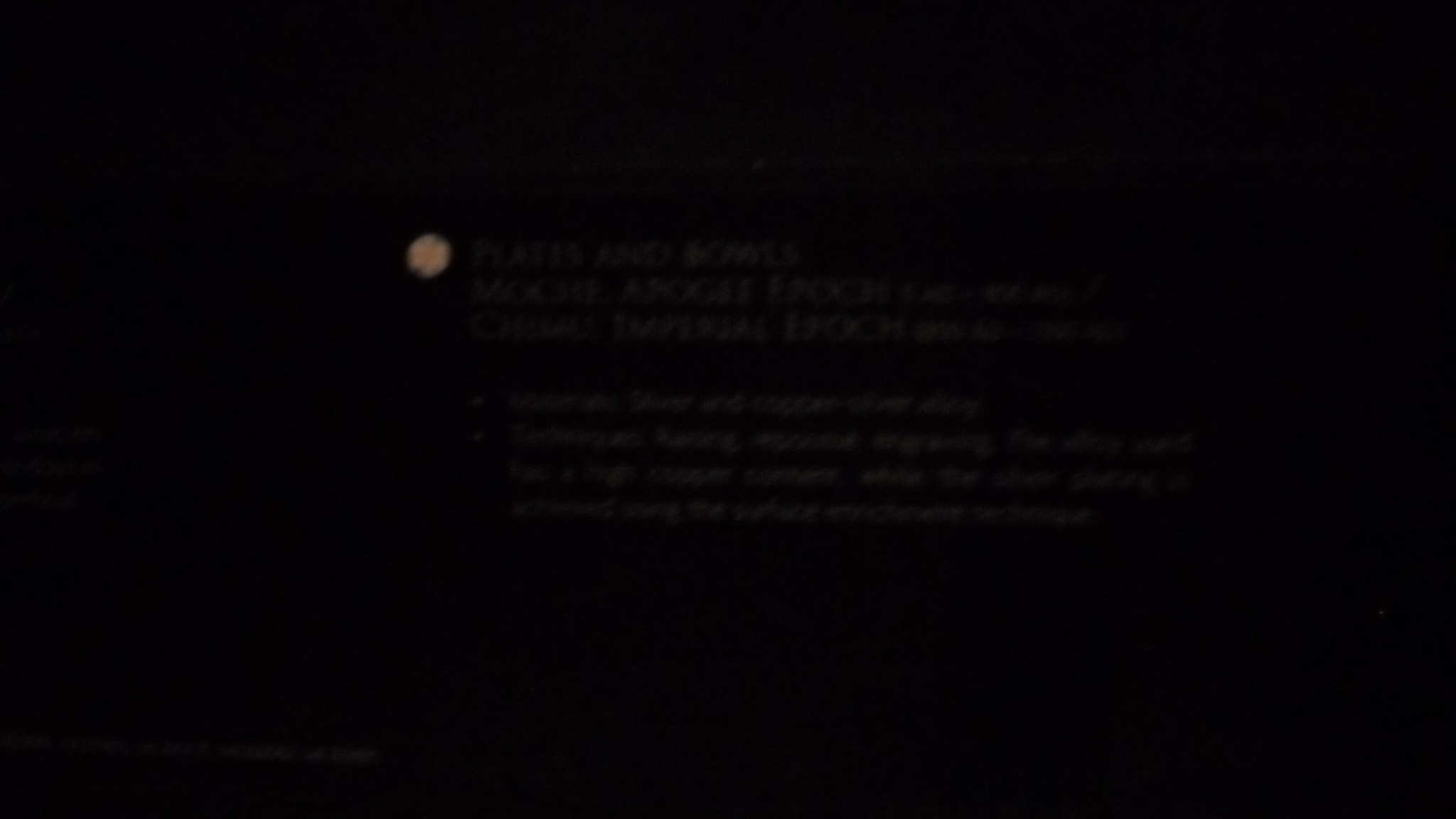This rectangular image, oriented with its longer sides running horizontally, predominantly features a black background. Near the center, slightly offset to the upper-left, is a small, light orange asterisk or star-like symbol. Adjacent to this symbol, beginning just to its right, is white text that spans horizontally across the image. The text is composed of seven lines, with the first three lines printed in a larger font than the subsequent four lines below them. Due to the overall darkness of the image, the text is difficult to decipher and might be in a different language. The remaining portion of the image is entirely black, contributing to its obscured and monochromatic appearance.